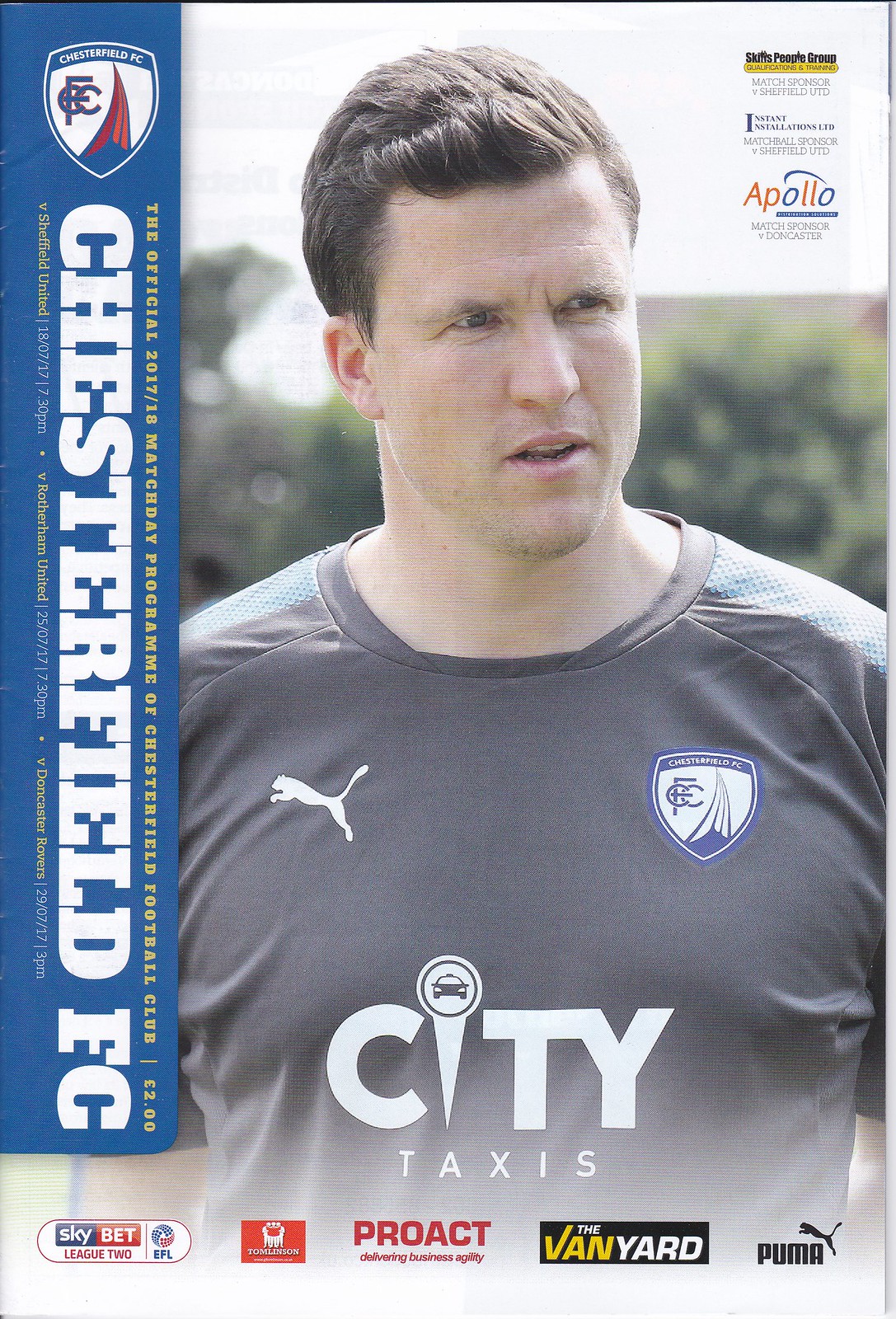This image appears to be the front cover of a Chesterfield Football Club match day program for the 2017-2018 season. Central to the cover is a photograph of a white male with brown hair, wearing a gray t-shirt. The t-shirt prominently features a white Puma logo on the upper right-hand corner, a Chesterfield FC shield logo on the left side of his chest, and "City Taxis" written in white across the middle.

The left side of the cover includes the Chesterfield FC shield logo with "Chesterfield FC" written beneath it. Situated at the upper right-hand corner are various company logos, including one that reads "Apollo," while the others are too small to identify. Additionally, the bottom of the cover showcases several more logos, including those of Sky Bet, League Two, EFL, Proact, The Vanguard, and Puma. The program cover features a vivid color palette of blue, white, red, orange, grey, yellow, black, and maroon. The overall layout suggests it is an official program likely distributed to attendees at Chesterfield FC football matches.